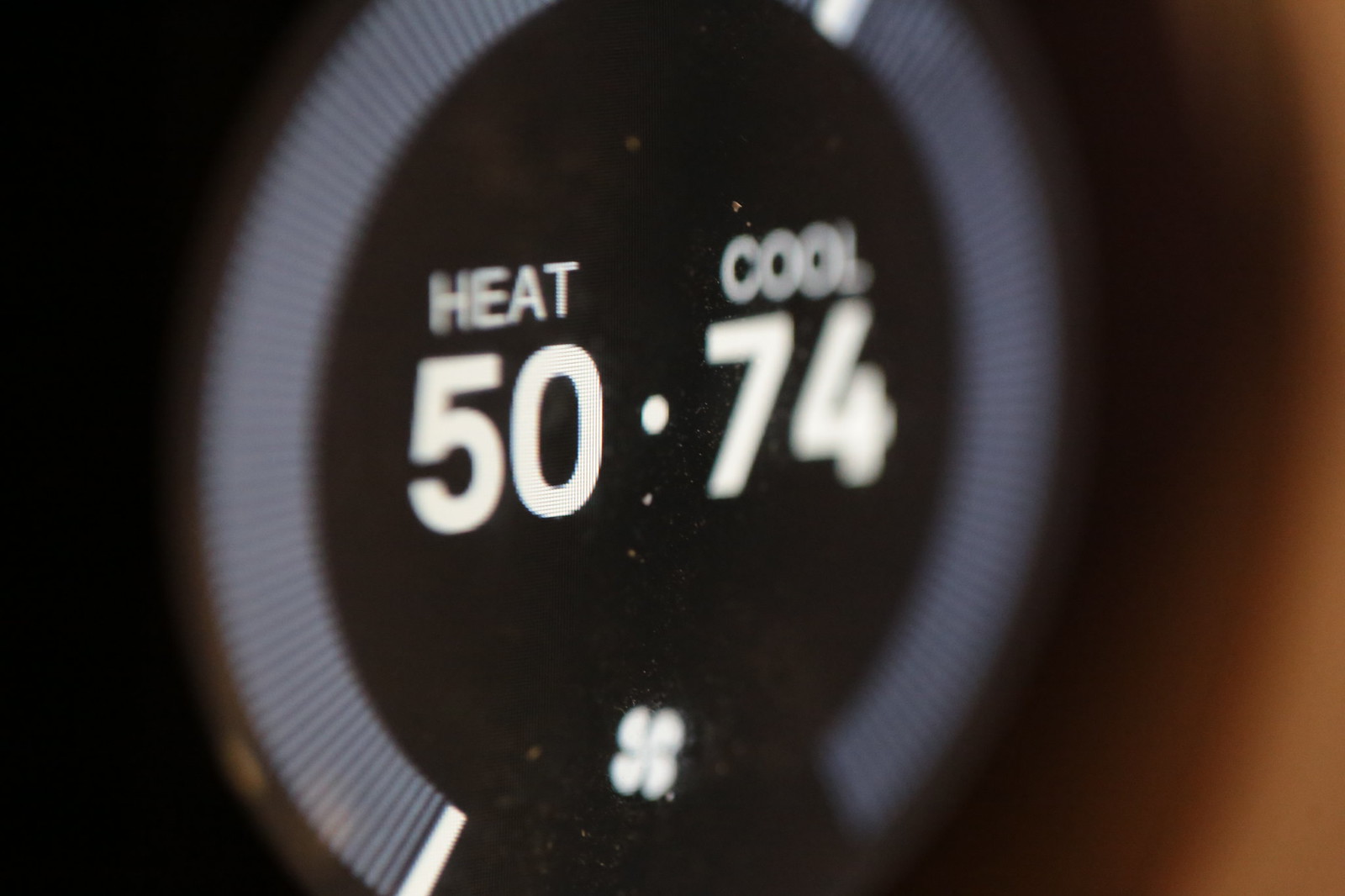In this out-of-focus, color photograph, presented in landscape mode, we see a digital display featuring a distinctive circular design. The ring, gray in color and adorned with horizontal ridges, is incomplete at the bottom, giving it a unique, open-ended appearance. Centrally situated within the gray ring is a contrasting black circle that hosts crucial information.

On the left side of the black circle, the word "HEAT" is displayed in capital letters, accompanied by a larger number "50" positioned below it, both texts clearer than their counterparts. To the right, the word "COOL" appears, followed by the number "74" in a larger font, though this part of the display is notably blurrier. At the very bottom of the black circle, there is an icon made up of four dots arranged in an overlapping square pattern.

The background of the image is heavily blurred, with a noticeable brown area toward the right side, adding to the overall indistinctiveness of the scene.